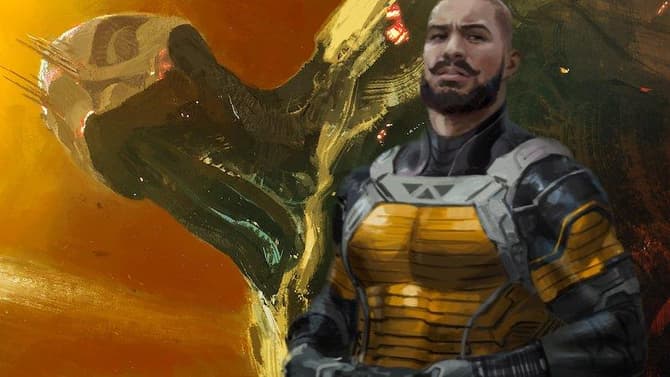In this detailed science fiction art piece, a bald man with white skin, a handlebar mustache, and a beard is depicted wearing an elaborate armored outfit. His gear consists of a chest plate and arm guards made of steel with a burnt brown color and gray trim, over a black shirt. He also seems to be wearing gloves. The man is looking sideways, appearing concerned, as if gazing at something in his peripheral vision. His attire includes yellow and gold stripes, adding to the ensemble's complexity and hinting at a superhero persona. Behind him, a larger image dominates the scene: a non-human, possibly cybernetic figure characterized by metallic green and gold colors. This figure, with a long, thick neck, two eyes, and a gold hat, looms mysteriously. The overall background of the artwork is washed out with hues of red and yellow, enhancing the dramatic and otherworldly atmosphere of the image.